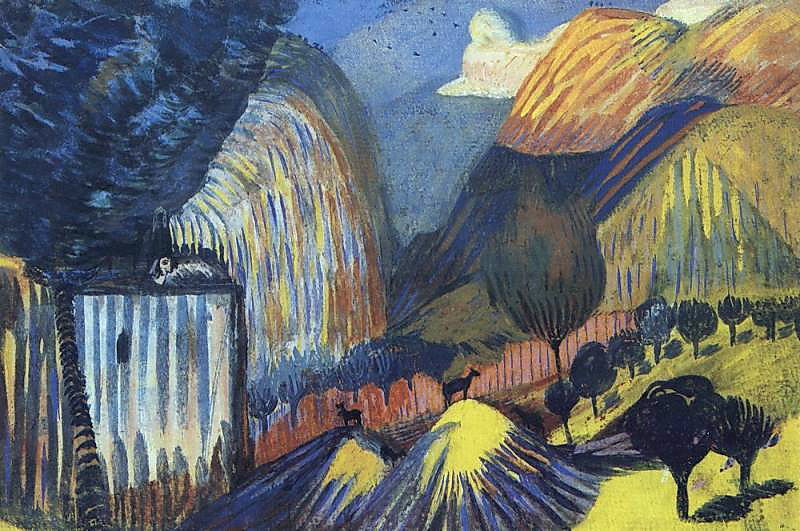This image depicts an impressionist painting of a vibrant landscape featuring a waterfall cascading through a valley surrounded by majestic mountains. The scene is imbued with a vivid palette of yellows, blues, light blues, dark blues, oranges, greens, and whites, accented by shades of beige and black. Thick brush strokes animate the terrain, creating a dynamic and textured view. In the background, the tall mountains with golden peaks rise to meet the sky, adorned with scattered clouds. A circle of birds flutters near the top center next to a cluster of blue clouds, adding life to the scene. The waterfall, positioned towards the middle left, flows gracefully down into the valley.

In the foreground, small hills dot the middle and bottom right, where four deer can be seen climbing. The valley is also characterized by two rows of trees, primarily green and black, adding depth to the landscape. A practical, man-made tower stands to the left, potentially a water diversion structure. To the right, a tall cliff fringed with trees adds a dramatic edge to the serene setting. This painting, devoid of any text, captures the natural beauty and tranquility of the landscape with a rich and intricate depiction of the elements.